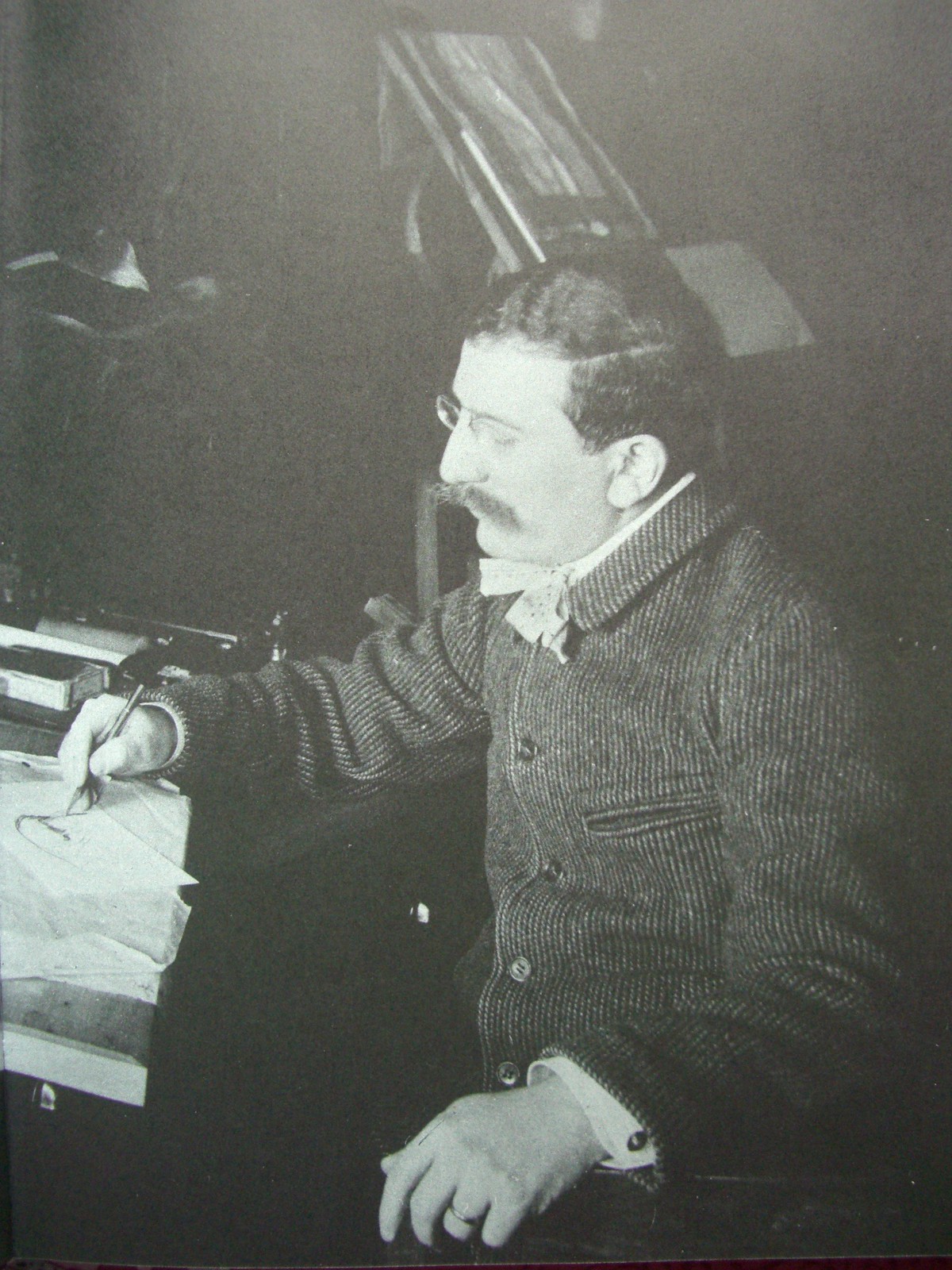This black-and-white photograph, marked by its old-fashioned and somewhat dark appearance, showcases a man in a central indoor setting, working intently at a desk. The room's details are sparse due to the image quality, but it is evident that the man is the focal point. He is well-dressed, wearing glasses, with dark hair and a mustache, and sports a distinct outfit comprising a striped, tweed-like, button-down jacket, a collared shirt, and a bow-like tie of light color. A ring adorns his ring finger. 

Seated at an inclined drafting desk, the man is absorbed in drawing what appears to be an artistic rendering rather than text, possibly a cartoon. His serious expression is emphasized as he holds a pencil over the paper. The desk in front of him, positioned slightly left in the image, bears various indistinct objects. Behind him, a partially visible canvas with an unknown drape further sets the scene. The entire image, devoid of any visible text, relies on its grayscale tones—ranging from white to multiple shades of gray—capturing a candid, timeless moment of concentrated artistry.